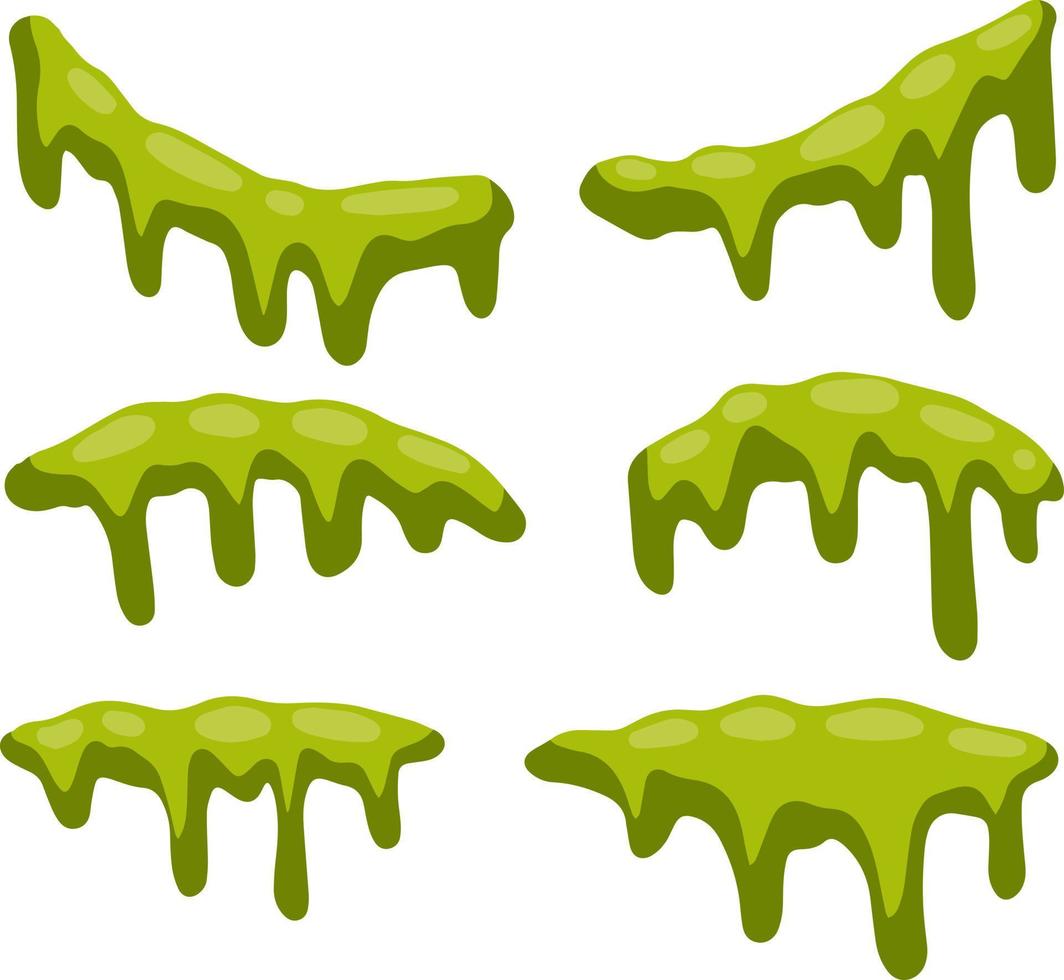The image features six distinct illustrations on a pure white background, resembling dripping blobs of green paint or slime. Each blob has a dark olive green outline with a lighter chartreuse green filling, which further contains several oval-shaped patches of an even lighter green. The blobs, appearing almost like dripping boogers, are arranged in two horizontal rows of three. Despite their similarities in shape and color, each blob is unique, differing in the number and length of drips extending from them. Some blobs exhibit drips curving downwards or upwards, while others display bumpy, irregular drip patterns. The crisp, sharp edges of the blobs give them a clip-art quality, as if they could be easily copied and pasted from the background.